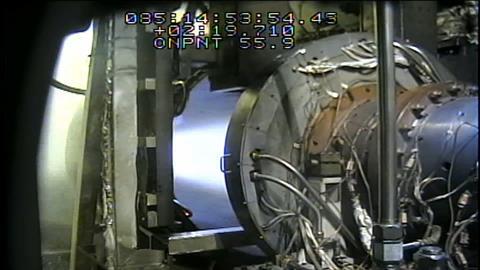The image is a small, grainy, wide, rectangular snapshot, likely from an industrial setting or factory. At the top, digital numbers are displayed in white with a black outline, possibly a timestamp, reading "085, 14, 53, 54, 48," followed by "+02, 19, 710," and below, "ONPNT 55.9." Dominating the right side and central area is a large, thick, circular steel apparatus with a giant tube attached to it. Numerous silver wires and cords extend from this metallic structure in various directions. A distinct black pole stands in front of it, cutting through the industrial chaos. The machine appears to emit a very bright white streak or laser beam from within the tube, illuminating its core. The left side is cluttered with additional mechanical components, including what might be another pipe, reinforcing the heavily industrial and mechanical nature of the scene.